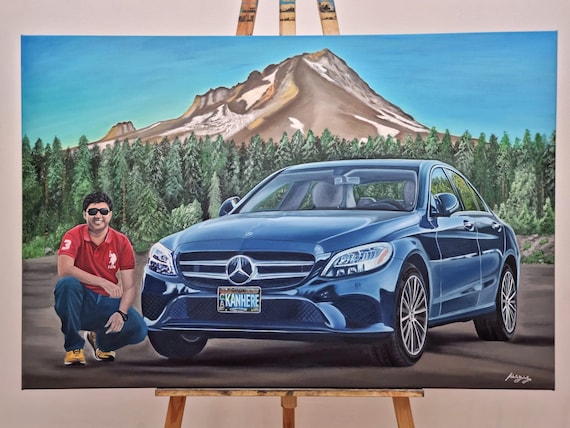This detailed image captures a traditional painting displayed on an easel set against a beige wall. The painting, executed with vivid colors, features a man positioned on the left side, dressed in a red polo shirt, blue jeans, and yellow sneakers, with sunglasses shielding his eyes. He is kneeling down and smiling beside a shiny, dark blue Mercedes-Benz, identified by its prominent silver grille and a license plate reading "KANHERE." The car’s interior appears gray. In the painting’s background is a lush row of pine trees displaying varying shades of green. Further back, a majestic, brown mountain with patches of white, suggestive of snowcapped peaks, rises against a clear blue sky. The foreground of the painting depicts light and dark green terrain, completing the scenic composition.